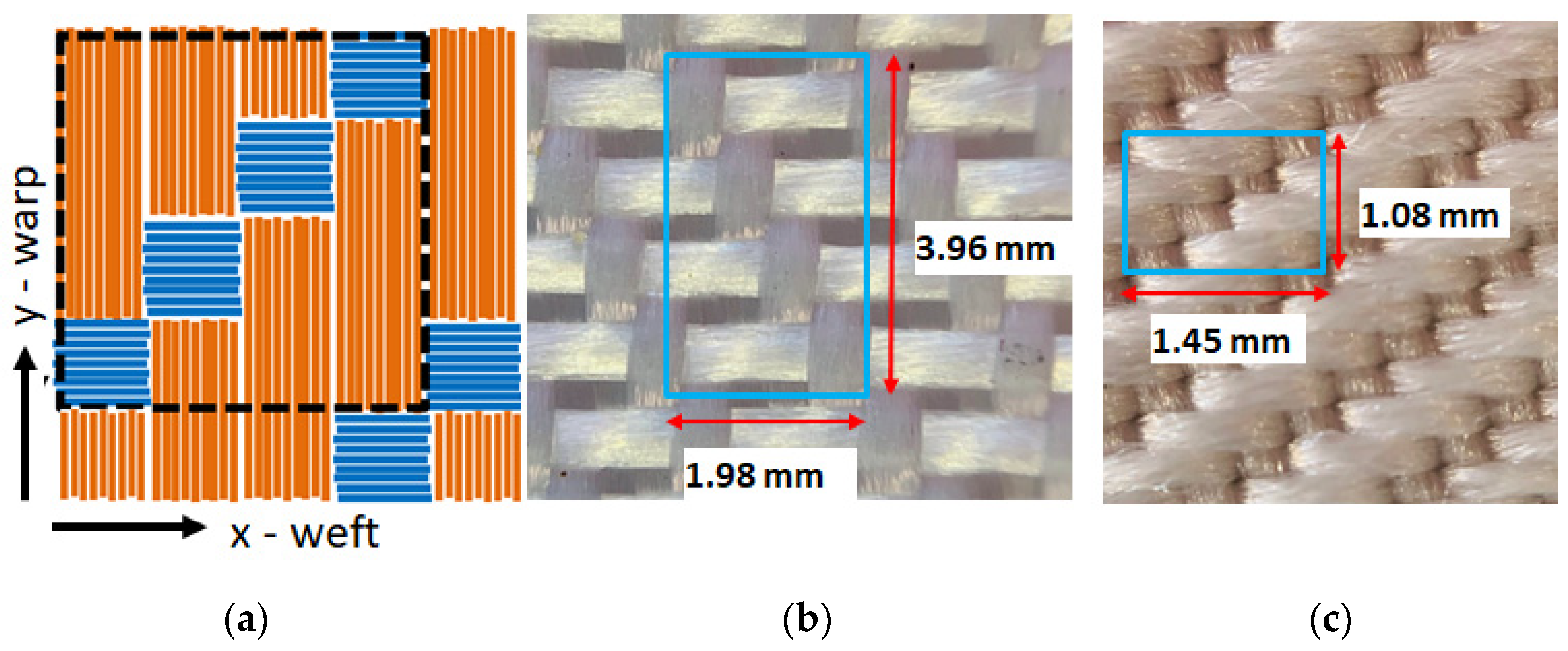The image consists of three distinct and detailed diagrams, each labeled A, B, and C in parentheses, showcasing different weaving patterns and measurements. 

**Diagram A** presents a pattern with vertical orange lines intersected by horizontal blue squares. In the top left corner lies a black square. Arrows are pointing upwards and to the right, labeled "Y-WARP" and "X-WEFT," respectively, indicating the warp and weft directions of the weave.

**Diagram B** is a close-up of a gray woven fabric, featuring a blue rectangle in the middle. It is measured with red arrows indicating dimensions of 3.96 millimeters in height and 1.98 millimeters in width, and the diagram is labeled with a B in parentheses.

**Diagram C** shows an even closer view of an off-white woven fabric, characterized by another blue rectangle. It measures 1.08 millimeters in height and 1.45 millimeters in width, and is labeled with a C in parentheses.

Each diagram provides intricate details on the structure and measurements of different woven fabrics, emphasizing the fabric's construction and precise dimensions.